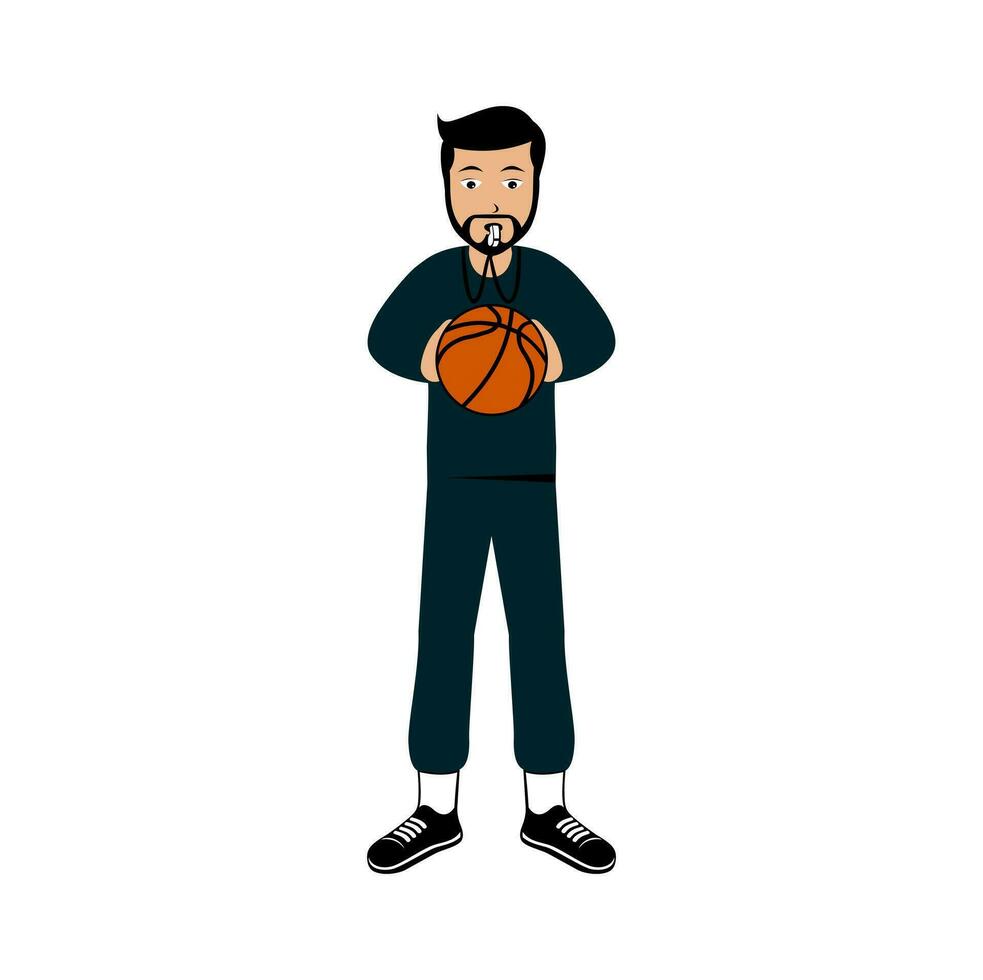This image showcases a cartoon figure of a man against a white background, dressed in a dark blue matching sweatsuit—comprising a long-sleeve shirt and pants that don't fully reach his ankles, revealing white socks. He has black sneakers with white laces on his feet. The man, who appears tall with notably long legs, holds an orange basketball with both hands extended in front of him. His dark hair is styled in a swoosh, and he sports a goatee. A referee's whistle, attached to a lanyard, hangs from his neck and is currently in his mouth. The figure looks down at the basketball, appearing serious and poised to demonstrate a throw, conveying a sense of readiness and focus. The detail in his serious expression and attire, combined with the slightly comical appearance of his high-rising pants, adds a whimsical charm to the image.